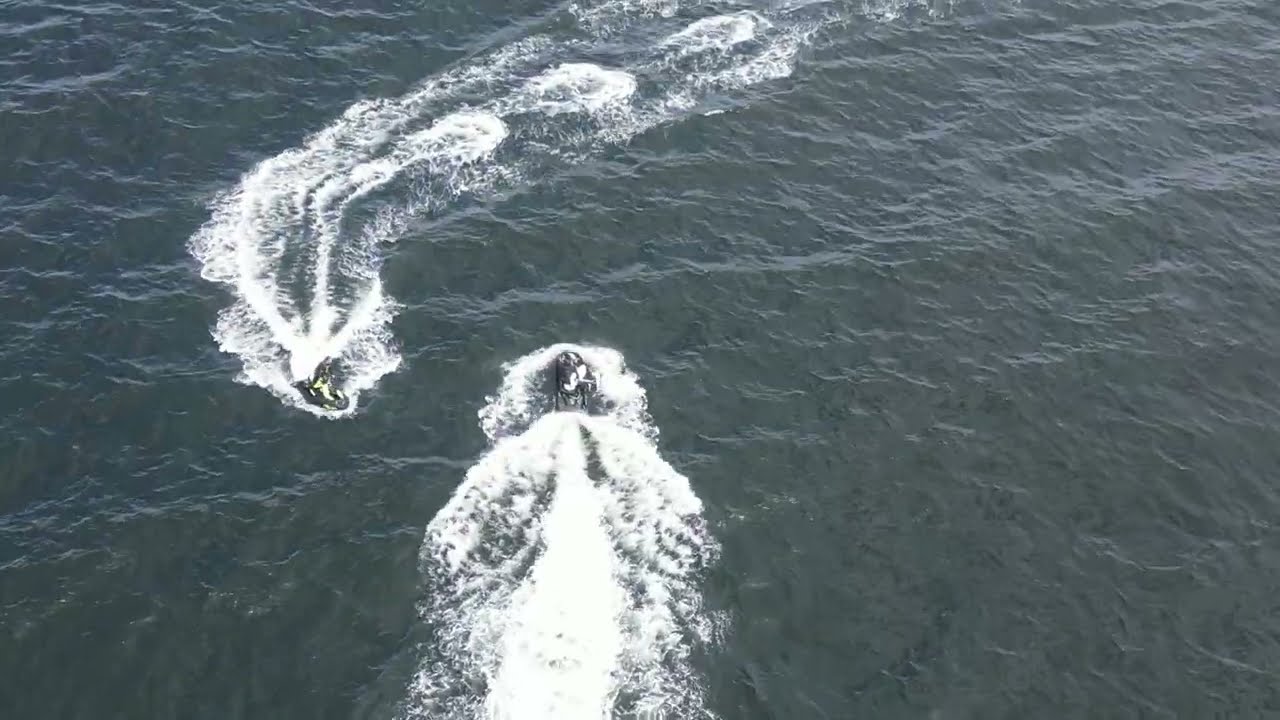An overhead photograph captures a dramatic scene over a dark greenish-gray ocean, likely on an overcast day. The water's surface appears slightly rough. Two large shapes, initially resembling fast-moving boats with big white wakes trailing behind them, surge through the water, one heading upward from the bottom of the frame and the other coming down at an angle from the top. Upon closer inspection, these shapes reveal themselves to be large whales, not boats, as evidenced by their size and the way they cut through the water. Both whales are moving swiftly towards each other, creating substantial waves and white foam in their wakes, suggesting a dynamic encounter in the ocean depths.